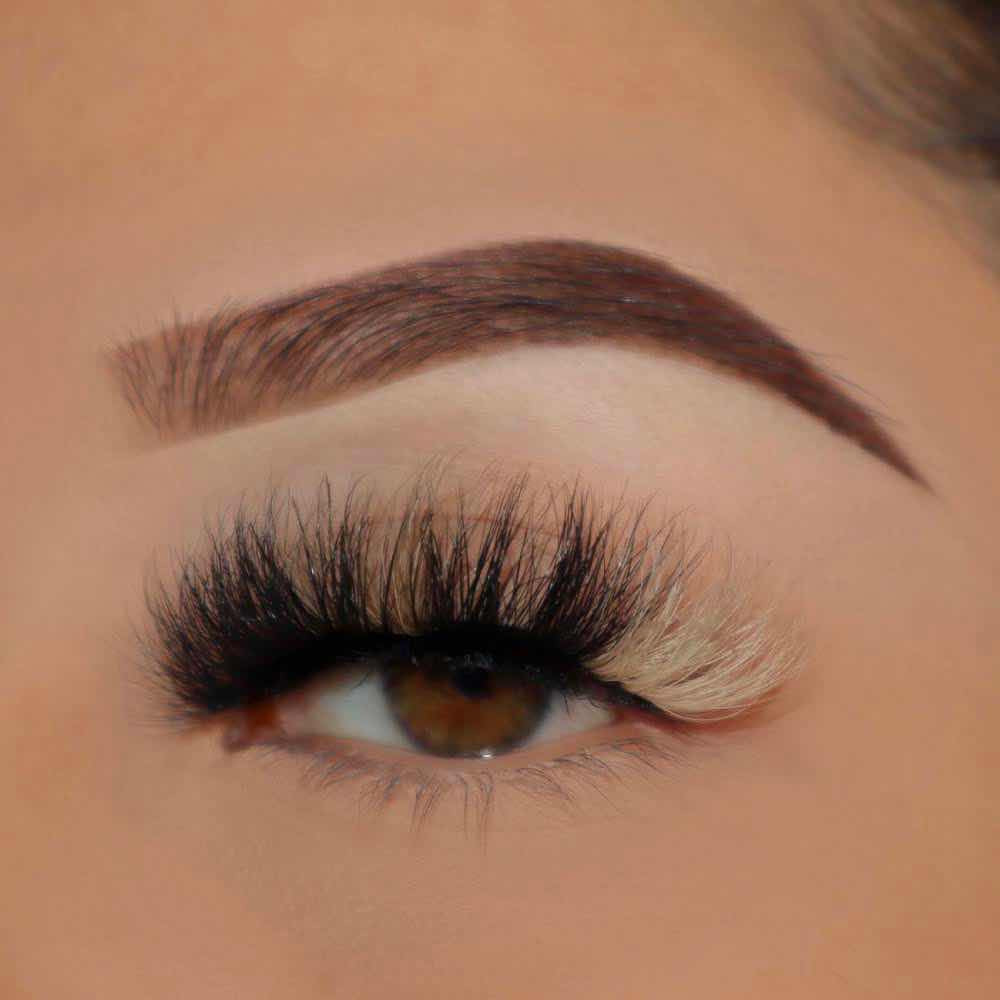This image is a close-up shot focused on a woman's left eye, capturing her features from just above the forehead to about an inch below her eye. The woman appears to have light, white skin and is likely in her twenties, inferred from her youthful skin. Her eye is distinctly brown, and the lashes exhibit a notable two-tone color pattern: approximately three-quarters of the lashes are black while the remaining quarter, on the inner side, is a striking blonde. Her eyebrow is meticulously manicured, appearing sparse but enhanced with precise, painted strokes that create a perfect, curved shape. This detailed grooming contributes to the overall intricate and beautiful presentation of her eye area.